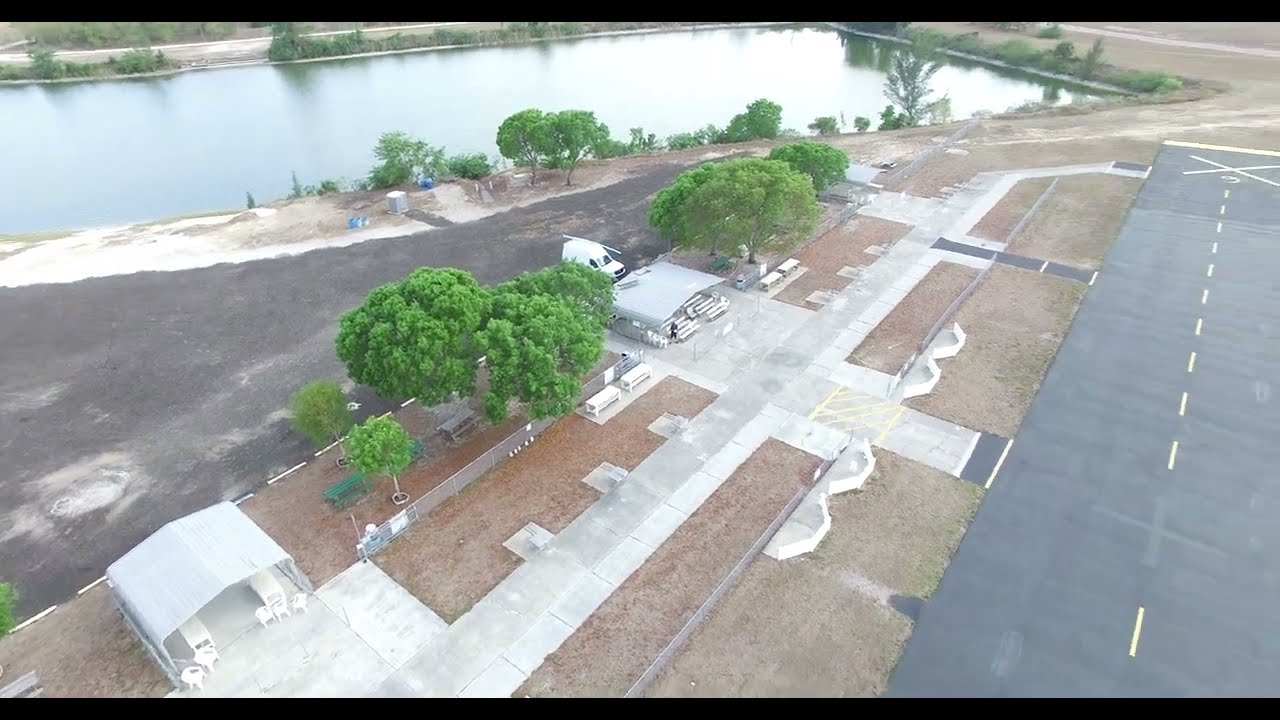This aerial photograph, presented in landscape orientation with horizontal black strips at the top and bottom, captures a meticulously maintained man-made environment. Dominating the upper section of the image is a greenish rectangular retention pond, bordered by greenery and reflecting nearby trees and hedges. On the right side of the frame, a road resembling a runway with a dashed line stretches vertically, culminating in a circular area marked with an X. Adjacent to this road, there is a paved pathway leading to several white-roofed, open-front storage shelters. These structures house various items, including vehicles, with a couple of vans parked behind them and chairs placed between the shelters. The area surrounding these paved pathways is predominantly brown dirt interspersed with a few trees and additional parked vehicles. A dirt road can be seen near the pond on the left-hand side, adding to the intricate layout captured in this detailed drone photograph.